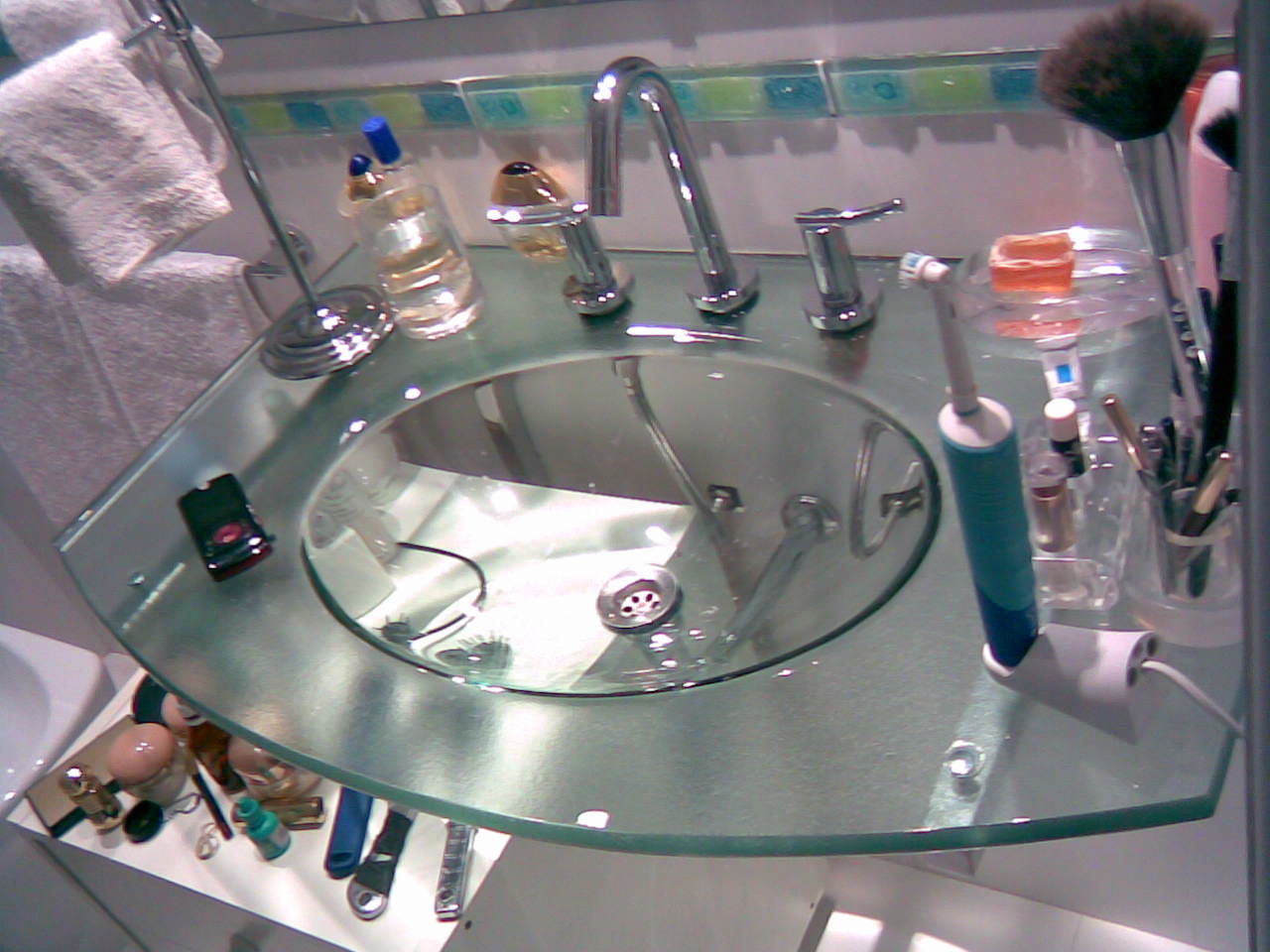In this image of a bathroom, the focus is on a modern, sophisticated sink setup. The sink bowl is entirely clear, giving it a sleek, minimalist appearance, while the surrounding counter space is made of frosted glass, which subtly reveals a blurred section of the area beneath it. On the counter, an electric toothbrush is seen charging next to a container holding an assortment of makeup brushes. A bar of soap rests beside two metallic handles used for controlling the water flow.

To the left, there are a couple of elegant perfume bottles and, at the corner near the bottom edge of the sink, a digital camera is casually placed. Adjacent to the sink station, a holder with either towels or washcloths hangs neatly. Below and to the left of the sink, another tier of counter space is cluttered with various makeup items, including jars, bottles, and several hairbrushes, reflecting a personal and everyday use of this modern bathroom.